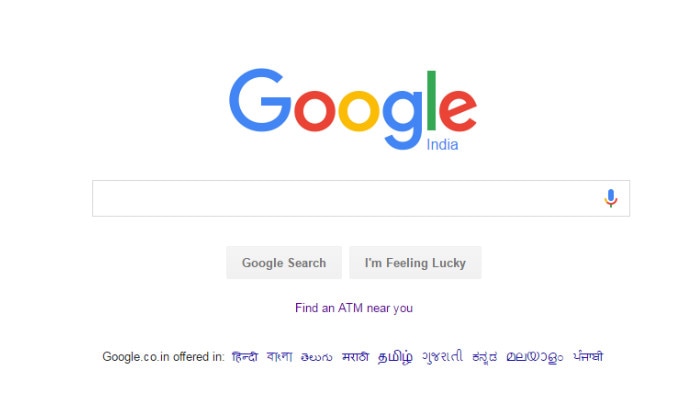Screenshot of the Google India homepage. In the center is the iconic Google logo, with a capital "G" in blue, followed by lowercase letters: a red "o", a yellow "o", a blue "g", a green "l", and a red "e". Beneath the logo, there's small blue text that reads "India." Below, a prominent white search bar stretches across the width of the page, featuring a microphone icon on its right end. Under the search bar are two gray rectangular buttons; the left one is labeled "Google Search" and the right one says "I'm Feeling Lucky". Further down, in purple text, it reads "Find an ATM near you". At the bottom of the page, the text "Google.co offered in" appears, likely followed by a list of language options.